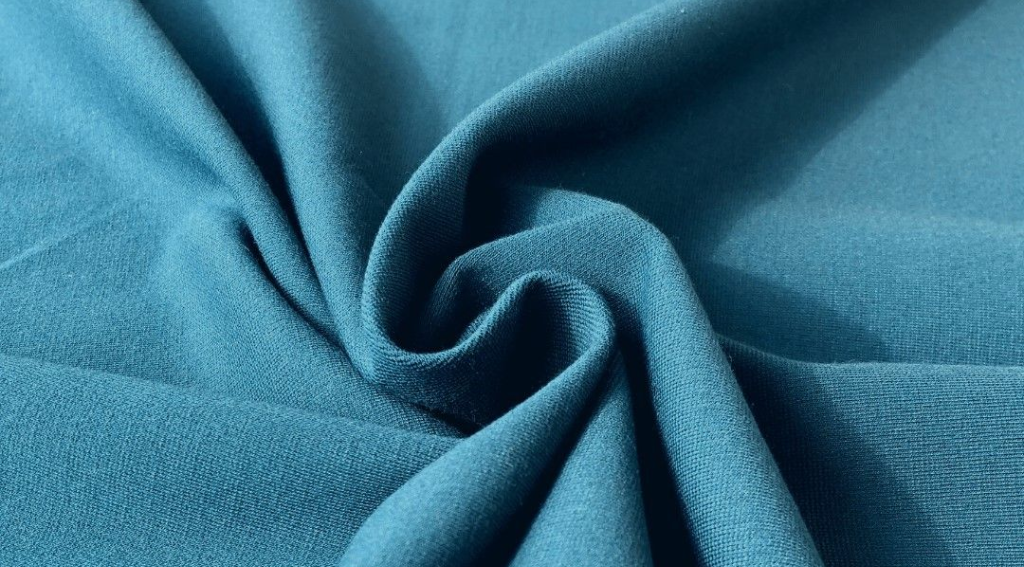The photograph captures a detailed close-up of a light to mid-blue cloth, resembling a blanket or curtain. The fabric is gathered into a central swirl, creating a rose-like or coiled appearance. This swirling bunched-up texture introduces shadows that emphasize the folds and enhance the three-dimensional effect. The cloth appears to be made of fine, likely cotton material and is visibly free from stains or imperfections, presenting a smooth, solid-colored surface without any patterns, borders, or threads. The image's zoomed-in perspective allows for a clear view of the lines formed by tiny holes across the fabric, further highlighting its pristine and fresh appearance.